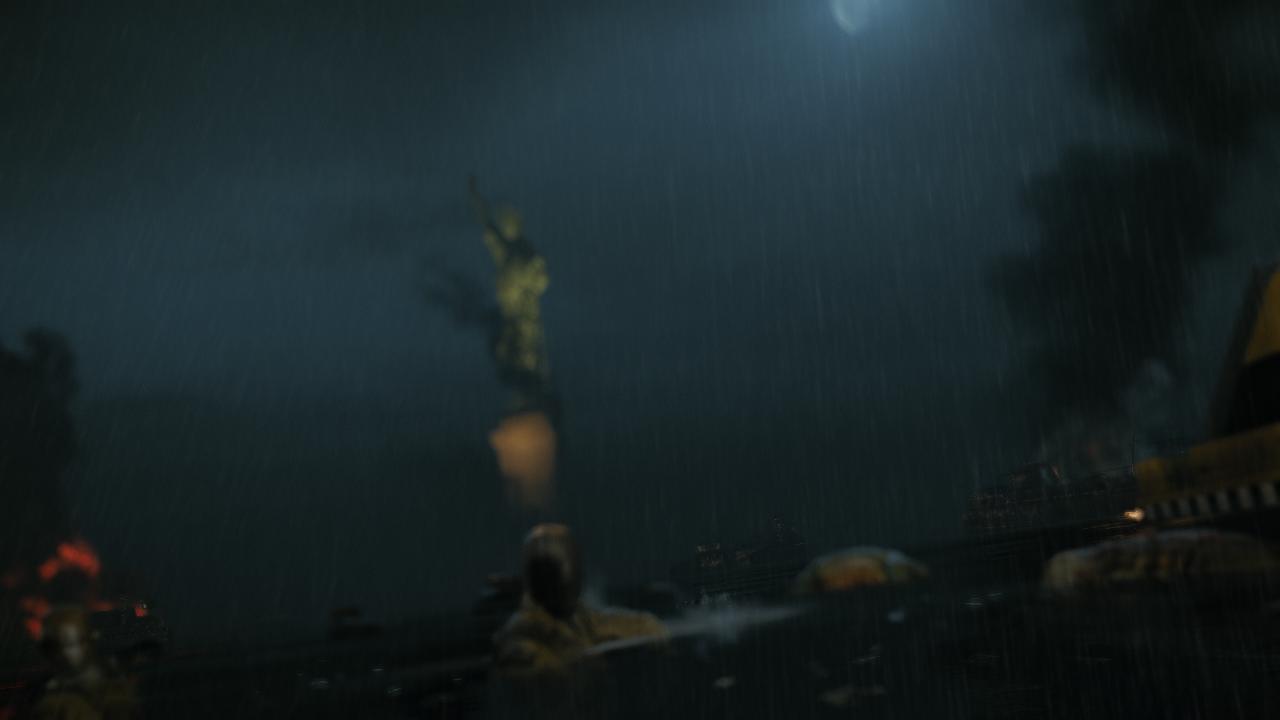In this detailed and atmospheric image, there is a dark and blurry scene, possibly from a video game or a museum exhibit, evoking a mysterious and somber ambiance. Dominating the center of the scene stands a statue, seemingly of a man, possibly an army figure, with a stone-like appearance. The background is cast in a deep, dark blue sky, faintly illuminated by the soft glow of the moon in the top right-hand corner. Rivulets of water ripple through the foreground, where soldiers or their remnants float alongside various debris, including bags.

To the far left, a building appears to be engulfed in flames, with a vivid red glow and billowing black smoke. Nearby, a metallic figure, possibly another statue, is silhouetted against the fiery backdrop, contributing to the chaotic and distressed environment. On the right side, more gray-colored buildings stand with smoke rising, but without visible flames, adding to the sense of destruction and ruin. Trees and a wall with slats appear faintly in the haze on the right, further accentuating the complexity and depth of the scene. This captivating and dark depiction captures a blend of natural and architectural elements, overshadowed by hints of fire and conflict.